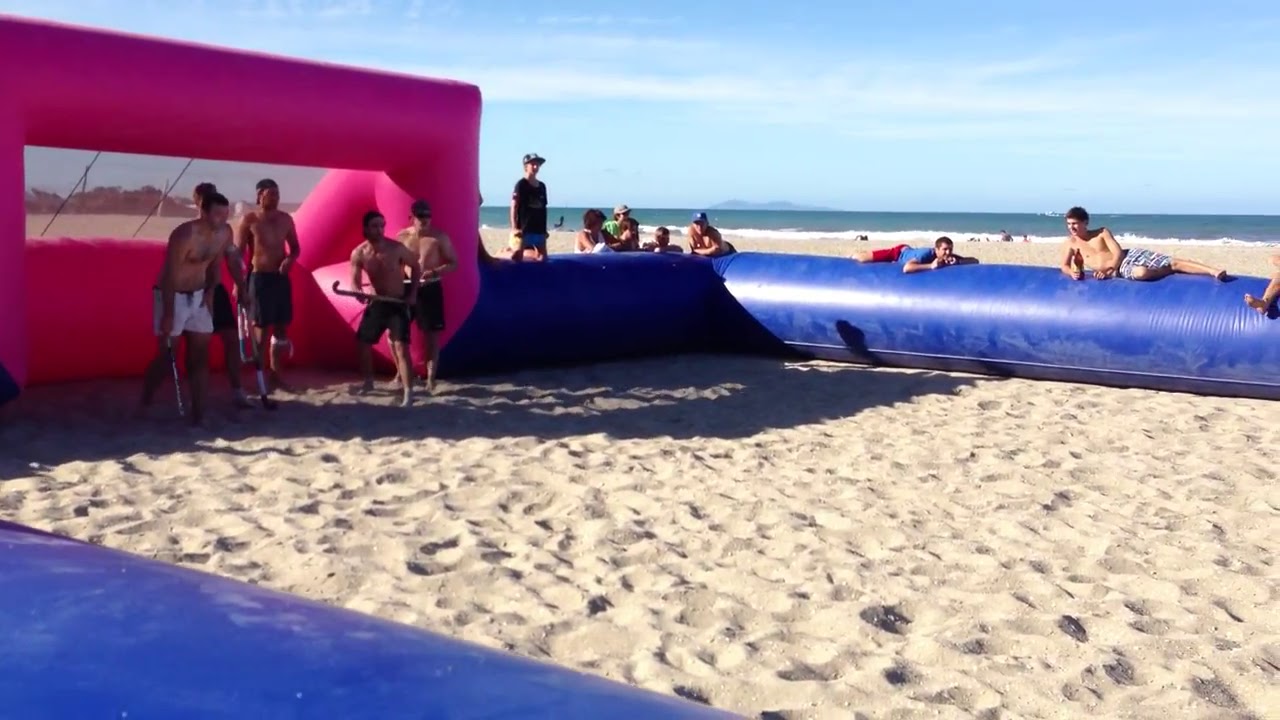The image captures a lively beach scene featuring a large inflatable sports field set up on a sandy shore, bordered by a vibrant blue perimeter with a neon pink goalpost at one end. Five shirtless men, donning beach shorts and sunglasses, stand at this end, clutching field hockey sticks, poised and ready to play a game. Surrounding the inflatable field, multiple spectators are seated and reclining against the blue inflatable edges, enjoying the scene. Some are even lying on the inflatable section, with one individual notably holding a beverage. Beyond this energetic gathering, the serene backdrop features more sand, the expansive blue ocean, and the clear, bright sky.